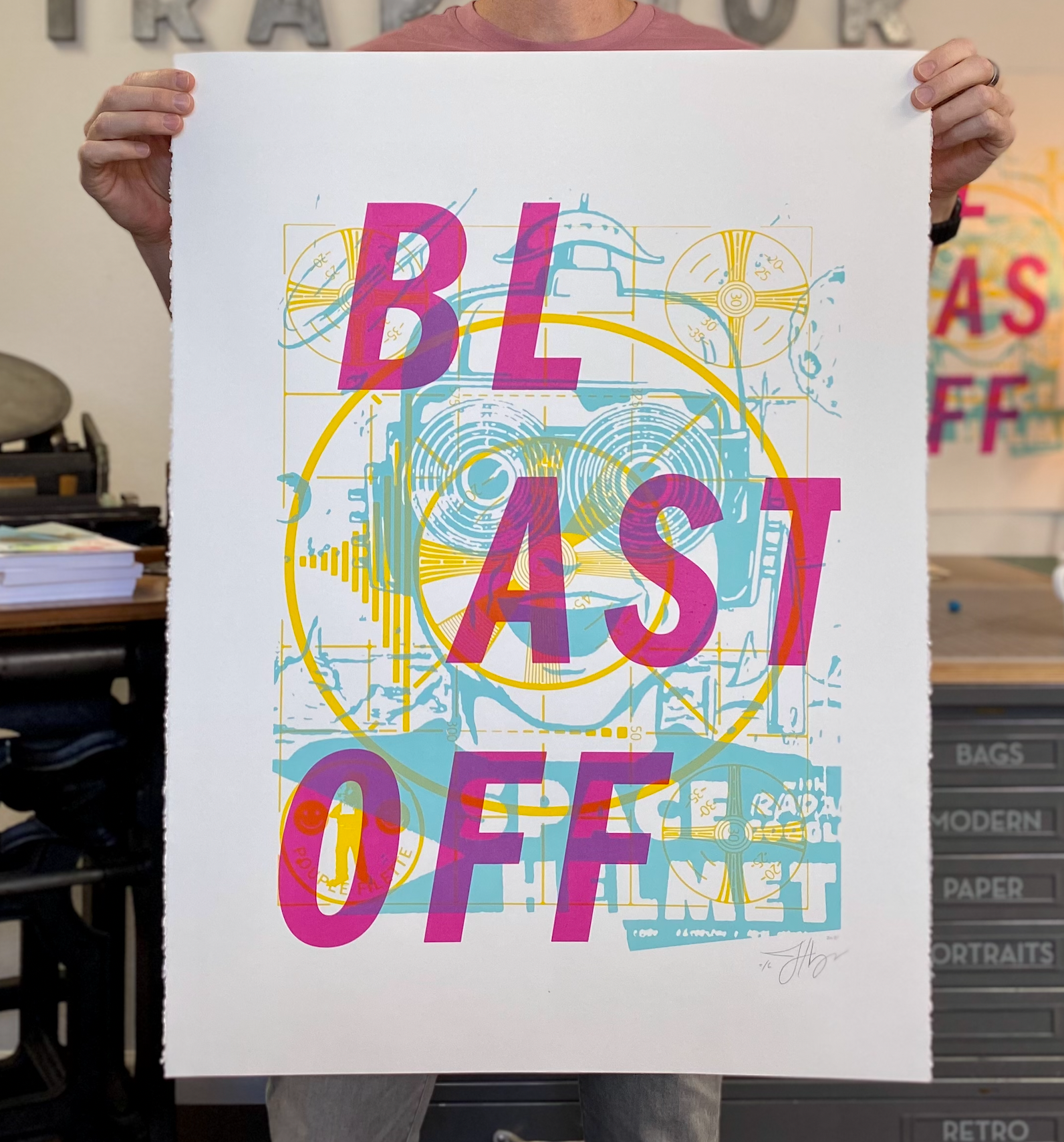In the image, a person is holding up a white poster with both hands, obscuring most of their body except for the tops of their shoulders, neck, and lower legs, which are clad in a pink collared shirt and pale blue jeans. The poster displays the phrase "BLAST OFF" in large, bright pink letters, segmented over three lines with "BL" on top, "AST" in the middle, and "OFF" at the bottom. A blue, whimsical illustration of a face wearing a vintage space helmet forms the backdrop of the text. This illustrated face features spiral goggles, a wide-open mouth with visible teeth, and yellow accents depicting radiating lines and circular designs evoking a playful, futuristic theme. Around the periphery of the poster, the setting appears to be a bustling print shop, marked by stacks of white papers, labeled drawers, and a mix of furniture with wooden tops and black legs. To the left, an office chair with a gray backrest is visible, adding to the industrious atmosphere of the space.